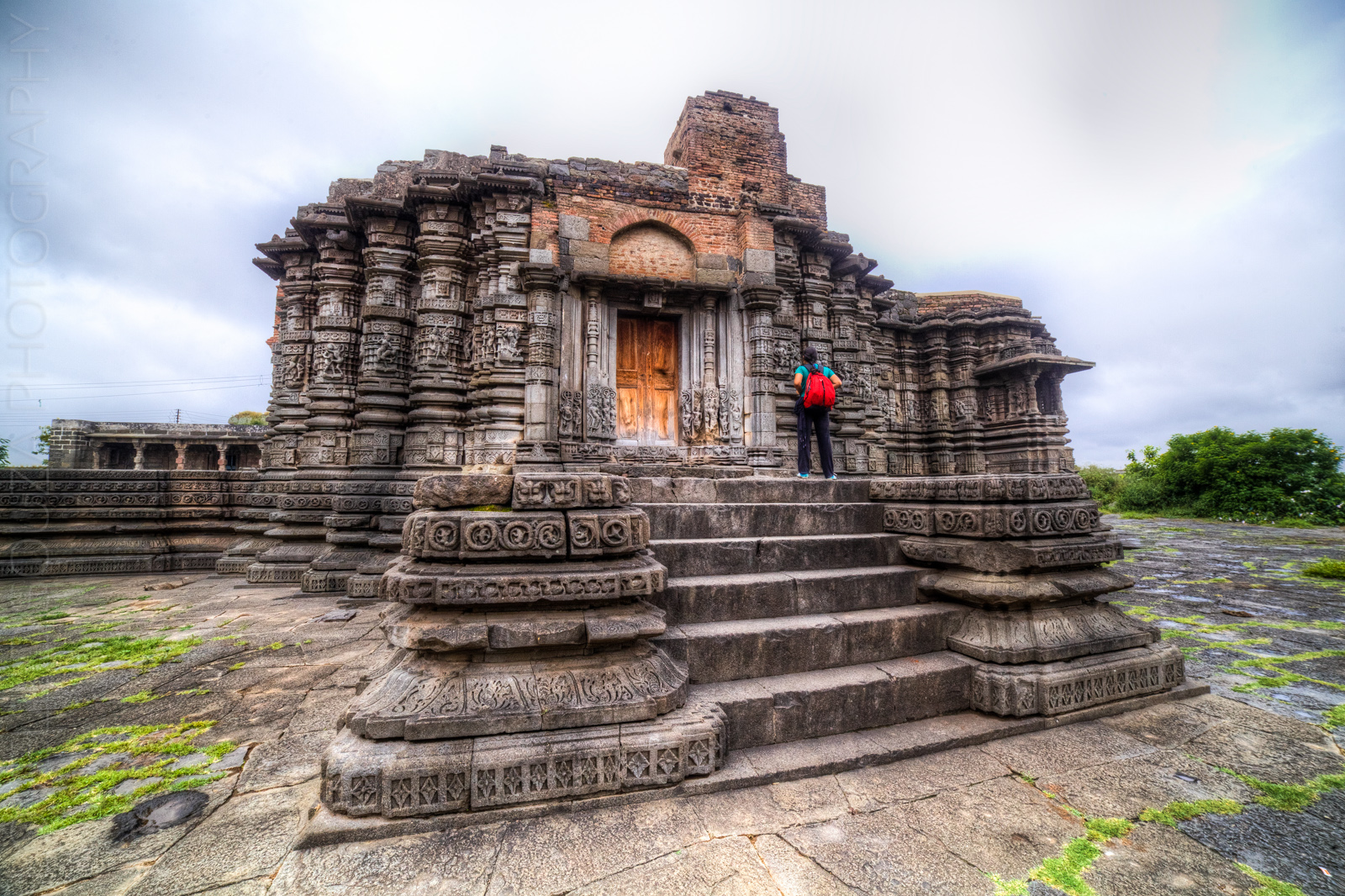In this captivating image of an ancient Hindu temple, intricate stone engravings and carvings adorn the weathered grey facade. A set of imposing stone steps leads up to a closed brown wooden door at the entrance. Climbing these steps, a tourist, identifiable by a red backpack, blue top, dark trousers, and blue shoes, carefully examines the elaborate carvings. The temple's architecture, featuring thick columns with layered ridges and a protruding brick tower visible over the main structure, speaks to its historical significance. This scene unfolds under a predominantly cloudy sky with patches of blue and white, adding to the allure of the setting. Surrounding the temple are stone pavements interspersed with patches of green grass, while a lush tree stands to the right, enhancing the temple's ancient and serene outdoor ambiance. The photograph, possibly taken with a wide-angle lens, conveys an artistic perspective, capturing both the grandeur and the minute details of this timeless structure.